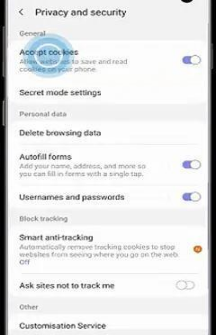A blurry screenshot of a webpage displayed on a cell phone screen, showcasing various privacy and security settings. At the top of the screen, there are options labeled "Privacy and Security" and "General." Below that, though not entirely legible, are settings for "Accept Cookies," with further details obscured by the blur. There are multiple sections indicated, each with toggle switches for different functionalities. These include options for "Secret Mode Settings," "Personal Data," "Delete Browsing Data," and autofill forms with fields for adding your name, address, and more to fill forms with a single tap. Toggle switches corresponding to "Usernames and Passwords" are turned on, while "Block Tracking" and "Smart Anti-Tracking," designed to automatically remove tracking cookies, are off. Additionally, a setting labeled "Ask Sites Not to Track Me" also has its toggle switch set to off. The screenshot captures the customization service details at the bottom, providing a comprehensive overview of the device's privacy and security features.